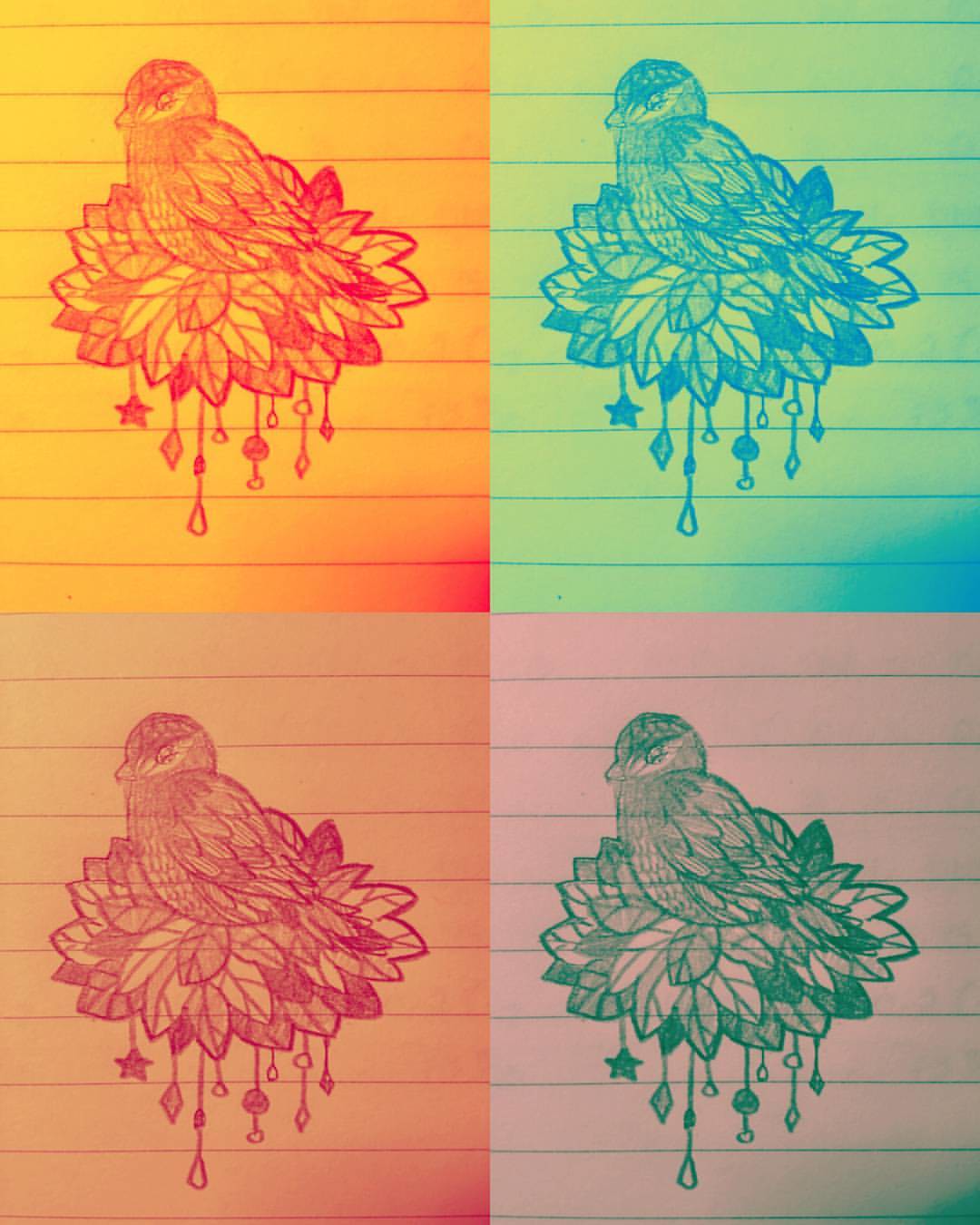This pop art style image features a detailed drawing of a bird resting in a nest of oval-shaped leaves, rendered in four distinct sections. Each panel reproduces the same intricate sketch with varying bright color filters, enhancing the visual diversity. The bird, facing right, is characterized by a shorter beak, a darker cap, and a dark eye, with finer feathers on its chest and slightly larger ones on its wings. The nest is composed of leaves with visible veins, all radiating outward from the bird. Decorative elements hang from the nest, including stars, diamond shapes, teardrops, and beads.

The panels are arranged as follows: the upper left panel showcases an orange filter with a red bird; the upper right panel features a greenish-yellow filter with a blue bird; the lower left panel is rendered in a reddish hue with a red bird; and the bottom right panel has a dark pink filter with a green bird. The entire image is set on lined paper, adding a unique texture and context to the art.